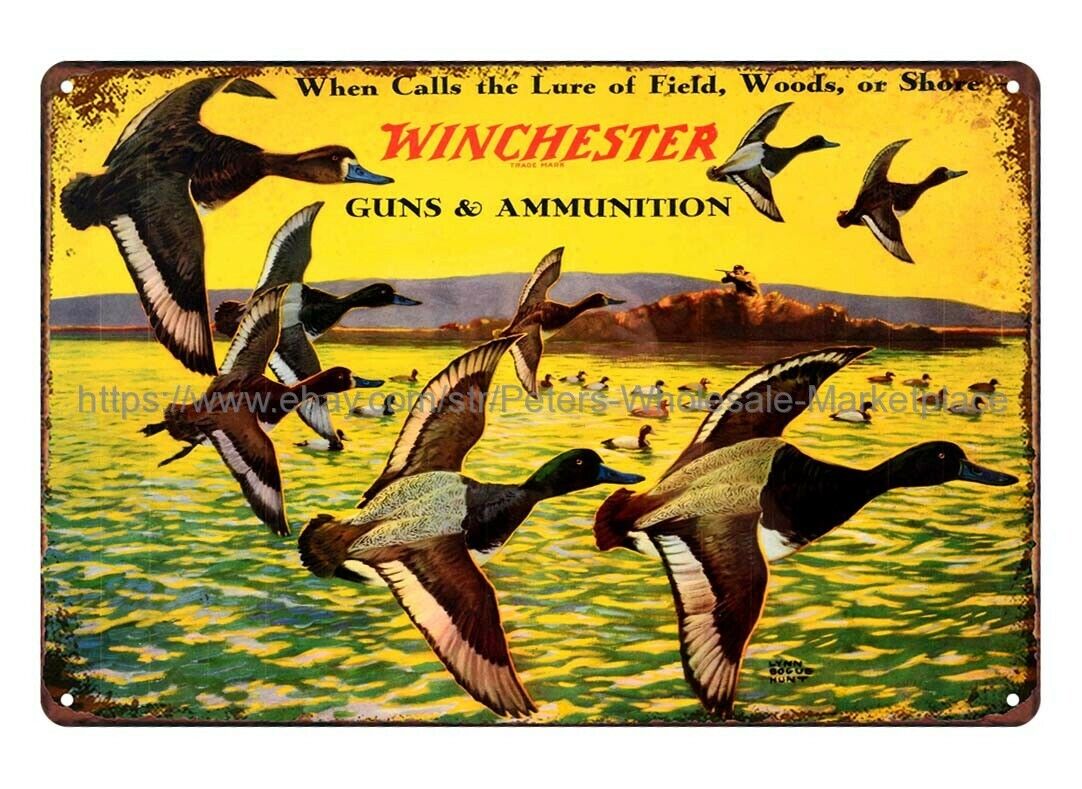This image is a vintage rectangular tin sign suitable for collectors, depicted in an advertisement style. The scene features a flock of mallard ducks in flight over a green and yellow lake, with the ducks displaying the characteristic green heads, brown bodies, white breasts, and wings. Among them, both male and female mallards are visible. In the background, additional mallards swim on the lake, all oriented towards the left. A hunter is positioned behind a brown blind, aiming his gun at the flying ducks. The sky above is a bright yellow, and textual details include the phrase "when calls the lure of field, woods, or shore" in black text at the top, followed by "Winchester" in red italics, and "guns and ammunition" in black text below that. The metal plate, intended for hanging, has pinholes in each corner. The overall color scheme prominently features yellows, greens, browns, and whites, adding to the nostalgic charm of the sign.